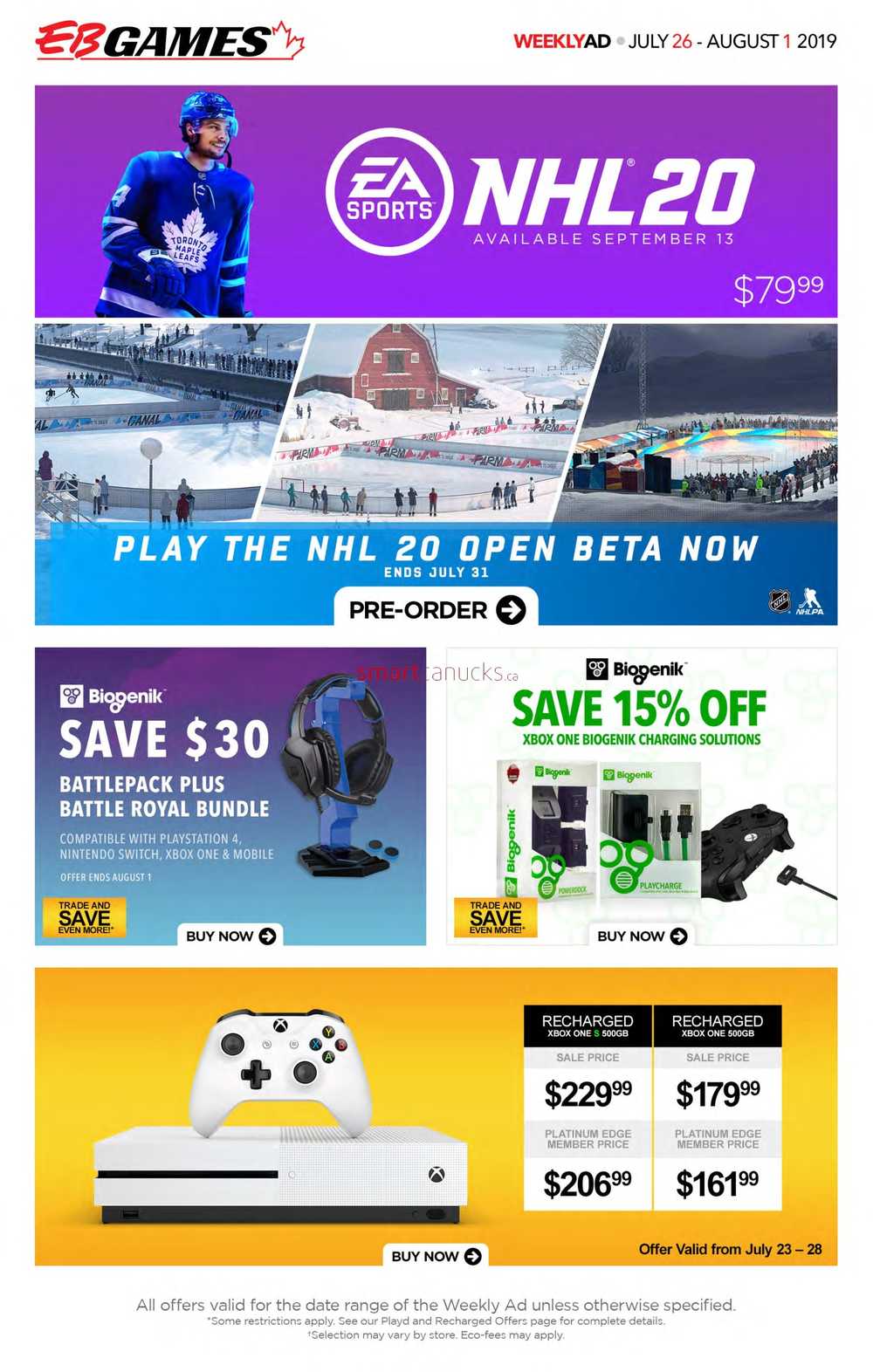This image is a detailed and colorful advertisement for EB Games, prominently featuring various promotions and offers. The ad is displayed in a rectangular, portrait orientation.

At the top of the screen, the background is white with the EB Games logo on the left, composed of "EB" in a stylized script and "Games" in bold black block letters. To the right of the logo, in smaller text, are the words “Weekly Ad” - with "Weekly" in red, "Ad" in black, followed by the dates "July 26 - August 1, 2019". Here, "July" and "August" are in black, while "26" and "1" are in red.

The advertisement is divided into four distinct horizontal panes:

1. **Top Pane (Purple Background):**
   - On the left side, a photo features a hockey player in a blue uniform.
   - Centered within the pane is an outlined white circle with "EA Sports" inside.
   - To the right of the circle, it displays “NHL 20 available September 13.”
   - The price "$79.99" is positioned in the bottom right corner of this pane.

2. **Second Pane (Blue Background):**
   - This pane showcases three photos at the top, depicting various snowy scenes, including people walking, people outside a barn, people on roads, and surrounding a hockey rink.
   - Below these images, a blue band with white text reads, "Play the NHL 20 Open Beta Now."
   - In smaller white text, “Ends July 31” is indicated below the blue band.
   - A section in white with black text commands, “Pre-Order” alongside a right arrow.

3. **Third Pane:**
   - This pane comprises two squares side by side, both advertising Biogenic products.
     - **Left Square:**
       - It has a promotion stating, "Save $30 Battle Pack Plus Royal Battle Royale Bundle," displaying a photo of headphones on a stand.
       - Compatible with PlayStation 4, Nintendo Switch, Xbox One, and Mobile.
       - A “Buy Now” button is at the bottom.
     - **Right Square:**
       - On a white background with green letters, the text reads, “Save 15% Off Xbox One Biogenic Charging Solutions,” accompanied by images of the products in white boxes.

4. **Bottom Pane (Yellow Background):**
   - Features a photo of an Xbox One console with a white controller on top.
   - To the right, details for two different sales:
     - "Recharged Xbox One 500GB Sale Price $229.99, Platinum Edge Member Price $206.99."
     - "Recharged Xbox One 500GB Sale Price $179.99, Platinum Edge Member Price $161.99."
   - At the bottom right of this pane, it states “Offer Valid from July 23rd through 28th.”
   - Finally, the bottom of the page, on a white background, contains disclaimers about the validity of the offers, stressing they are only valid for the date ranges indicated.

This comprehensive advertisement from EB Games is packed with visuals and detailed information on special offers, making it a compelling promotional display.